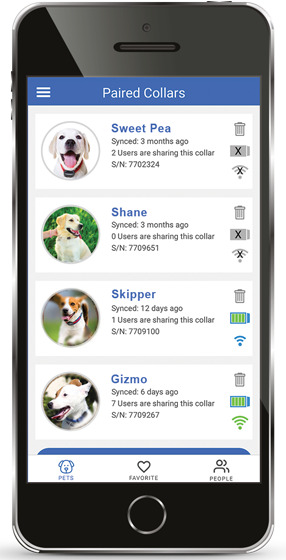The image depicts an older model iPhone displaying a screen with multiple sections detailing various dogs and their associated collars. At the top of the screen, there's a blue banner labeled "Paired Collars," with a navigation menu on the left side. 

1. The first section features a dog named Sweet Pea. A photo of Sweet Pea shows her with an open-mouth smile. The text indicates that her collar was synced three months ago, and it is being shared by two users. The serial number SN-770-2324 is listed. There are icons including a trash can, an 'X' indicating a disabled battery, and an 'X' over the Wi-Fi symbol suggesting no signal.

2. The second section showcases a dog named Shane. The image of Shane is accompanied by details stating his collar was also synced three months ago, but it has no users sharing the collar. The serial number is SN-770-9651. Similar to Sweet Pea, there is a trash can icon, a grayed-out battery with an 'X,' and a Wi-Fi signal with an 'X.'

3. The third section displays a dog named Skipper, who appears running in his photo. His collar was synced 12 days ago and is shared by one user. The collar’s serial number is SN-770-9100. This section has a trash can icon, but here the battery icon is full and the Wi-Fi signal icon is blue, indicating active connectivity.

4. The final section features a dog named Gizmo. Gizmo's picture shows his collar synced six days ago and shared by seven users. His collar’s serial number is SN-770-9267. Like Skipper, the battery icon is full and the Wi-Fi signal is green, indicating strong connectivity. The trash can icon is grayed out.

At the bottom of the screen, there are three menu options labeled "Pets," "Favorites," and "People."